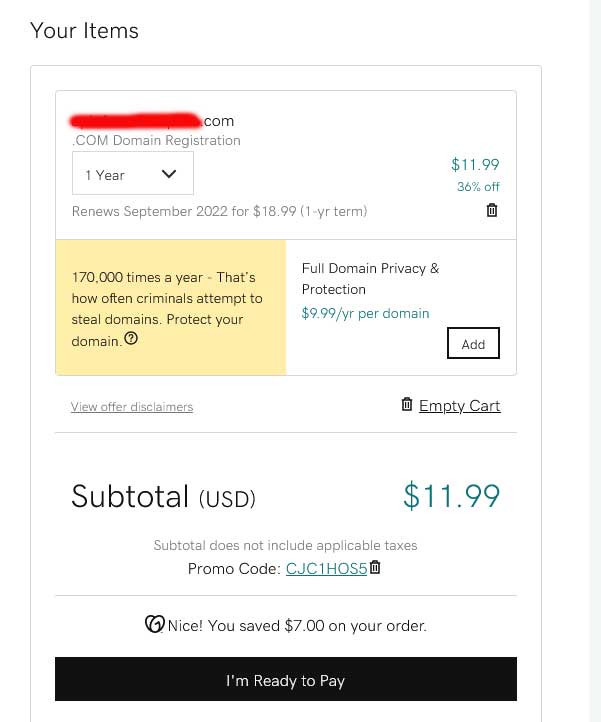This image captures the contents of an 'Items' window, detailing a domain registration purchase. At the upper left corner, the heading "Your Items" is displayed in black font. Beneath this, a thin gray outline frames a white box that contains specific details about the items listed.

Inside the white box, in the upper left section, a redacted line is visible, ending with ".com". Directly below, it reads ".com Domain Registration." Further down, a dropdown option shows "One Year," and to its right, the price is listed as "$11.99." 

Additionally, a note indicates a "36% off" discount below the price. Adjacent to these details, there is a small trash can icon for deleting the item. The subtotal is clearly marked as $11.99. Further down, a promo card highlights a savings of $7 on the order with a cheerful message, "Nice, you saved $7 on your order."